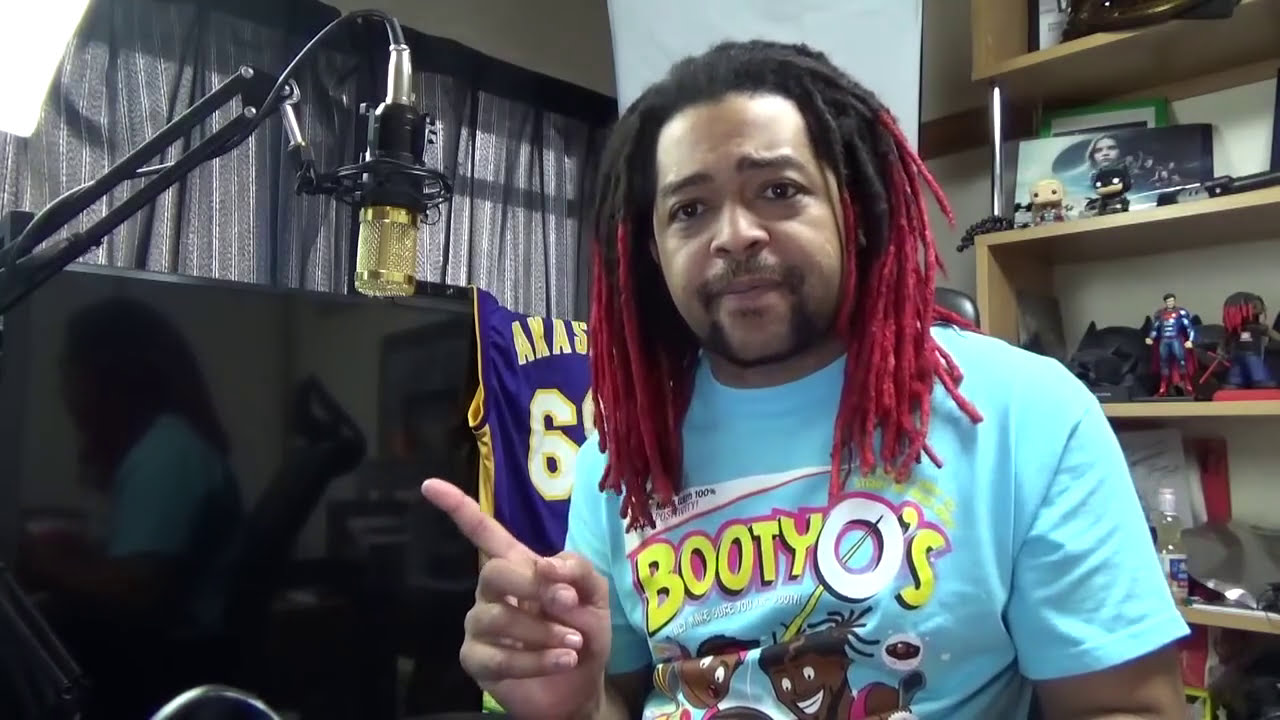This image captures an African-American man with dreadlocks that transition from brown to vibrant red at the tips. He has a full beard and mustache resembling a Fu Manchu style. The man is wearing a bright blue shirt with the text "Booty O's" in yellow and pink, featuring WWE characters. He is pointing his finger, possibly engaging in a recording or podcast session, with a black and gold microphone visible to the left of his face.

The background includes a Los Angeles Lakers home jersey with the number 6, partially obscured by letters like "AKAS." To his right, there’s a TV screen reflecting his image and a shelf displaying various items, including action figures like Superman and Batman, some Funko Pops, and a bottle of liquid. Gray curtains hang in the room, contributing to the ambiance of a cozy recording space. The man’s expression, featuring a raised eyebrow, suggests he might be questioning something or making a point.